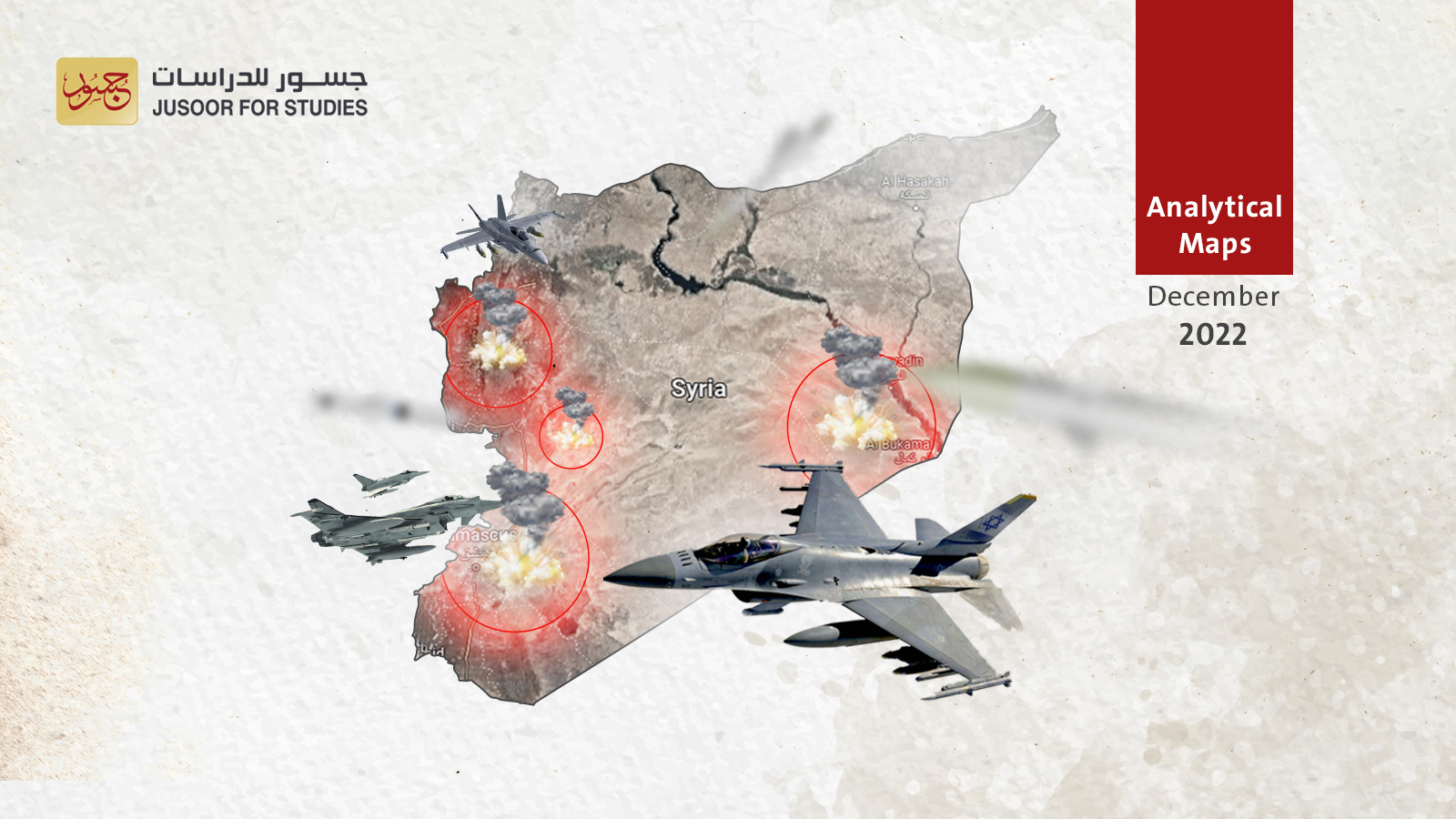The image is a highly detailed analytical map of Syria, set against an off-white background. A prominent red rectangle in the top right corner contains the title "Analytical Maps" in white letters, with "December 2022" written in black underneath. Within the map's boundaries, Syria is depicted in various shades of grey with a rocky texture. Numerous target areas, marked with red circles, indicate cities experiencing explosions, with dark gray smoke rising from fiery white-yellow bases. Several fighter jets, illustrated smaller than the country but quite detailed, are shown flying around the edges of Syria; three face eastward, while a larger jet in the foreground faces westward, all equipped with bombs. The upper left corner of the image features Arabic writing and a gold label with red lettering, translated below as "JUSOR for studies," spelled J-U-S-O-O-R. The overall composition of the map paints a grim picture of military activity within Syria, emphasizing areas under attack and the presence of fighter jets.